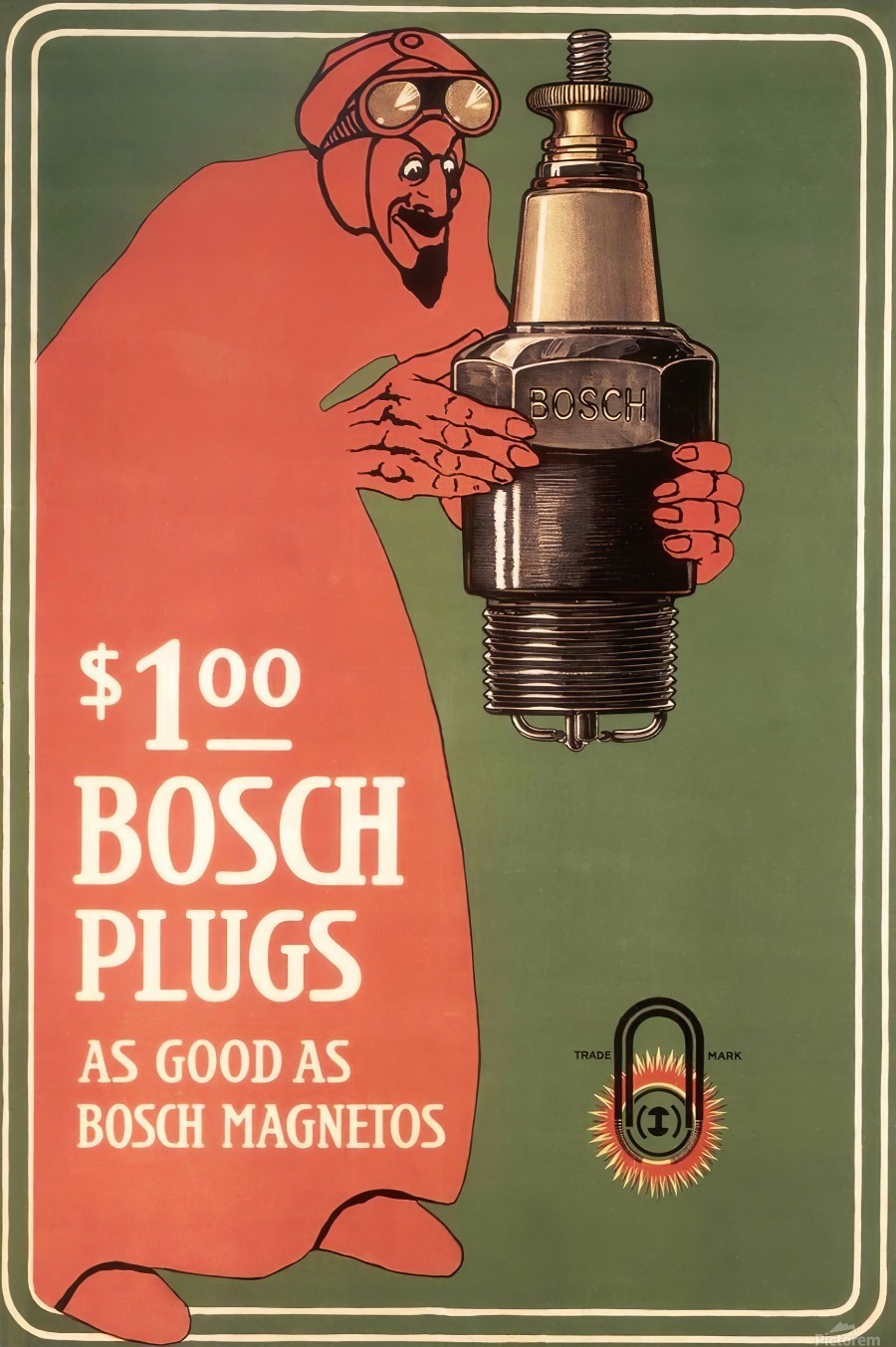This illustrated advertisement, likely from the late 1920s to the 1950s, features a vintage promotional style set against a drab olive green background. The image is bordered with thin white lines, framing the scene. Dominating the rectangular flyer is a bright orange-red, devilish figure depicted almost entirely in red, symbolizing the character of the devil. The figure has exaggeratedly large, detailed red hands extending from its long robe, complete with sharp red fingernails. His facial features include a sharp-pointed goatee, a mustache, white eyes with dark pupils, and a prominent nose. Atop his head are red steampunk goggles pushed up above his eyebrows, and he seems to be wearing a turban-like headpiece.

The devilish character is shown holding a spark plug prominently marked with the word "Bosch." The description of this plug highlights a screw-like base, a bolt in the middle, a golden section, and another spring-like element at the top. To the left of the figure, the advertisement text reads in white font: "$1 Bosch plugs, as good as Bosch Magnetos." At the bottom of the image is a depiction of a green-black lock with a red halo, indicating the trademark, enhancing the antique and mysterious vibe of the illustration.